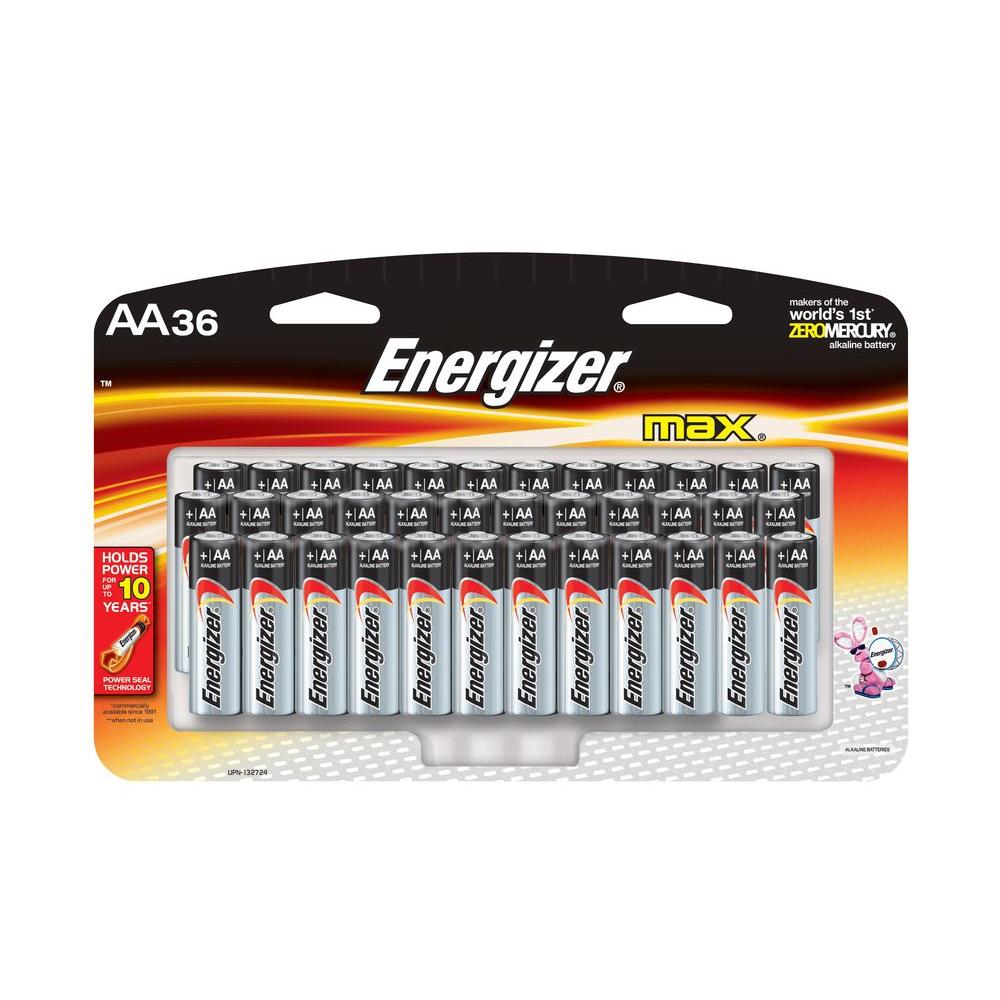The image features a package of Energizer Max AA batteries. At the top left corner of the package, "AA-36" is prominently displayed, indicating the quantity. On the top right, the text reads, "Makers of the World's First Zero Mercury," with "Zero Mercury" highlighted in yellow uppercase letters, and the following line, "Alkaline Battery," written in large but not all-caps letters.

In the center of the package, the brand name "Energizer" is boldly printed, followed by "Max" in yellow letters. Below this branding, there is a graphic representation of numerous batteries arranged in three rows. The first and third rows are offset to the rightmost side, while the middle row is shifted to the leftmost side of the package.

On the left side of the package, a box conveys the message, "Holds power for up to 10 years," underlining Power Cell Technology. To the right, an image of the iconic Energizer bunny can be seen, depicted as a pink bunny wearing sunglasses and beating a drum.